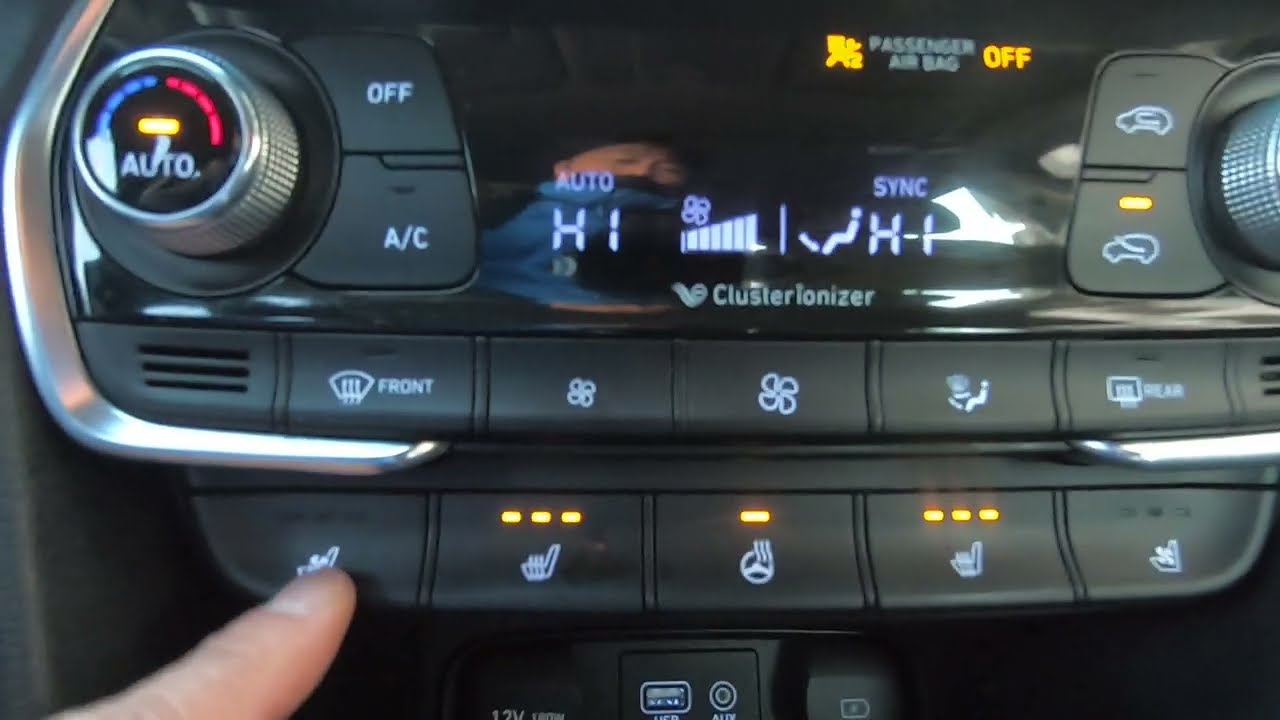This image showcases a close-up view of a car's central console, specifically its air conditioning control unit. An index finger at the bottom left is pressing a button on the control panel. The console features multiple buttons and displays: Starting from the top left, there is a circular knob with five blue squares on the left side and five red squares on the right side, with the word "auto" and an orange light at the center. To the right of this knob is a button labeled "off," and below it is another button that says "A/C." To the right of these buttons, there is an electronic display showing "auto high" in white font. Adjacent to this display are multiple bars with a fan symbol, and further to the right, it says "sync high." Additionally, there are other controls for the car’s heating, air conditioning, defroster, and airflow direction, although these specific details are not visible in the image. The console appears to be well-equipped, and aspects of the stereo system are seen with various indicators showing the current settings.